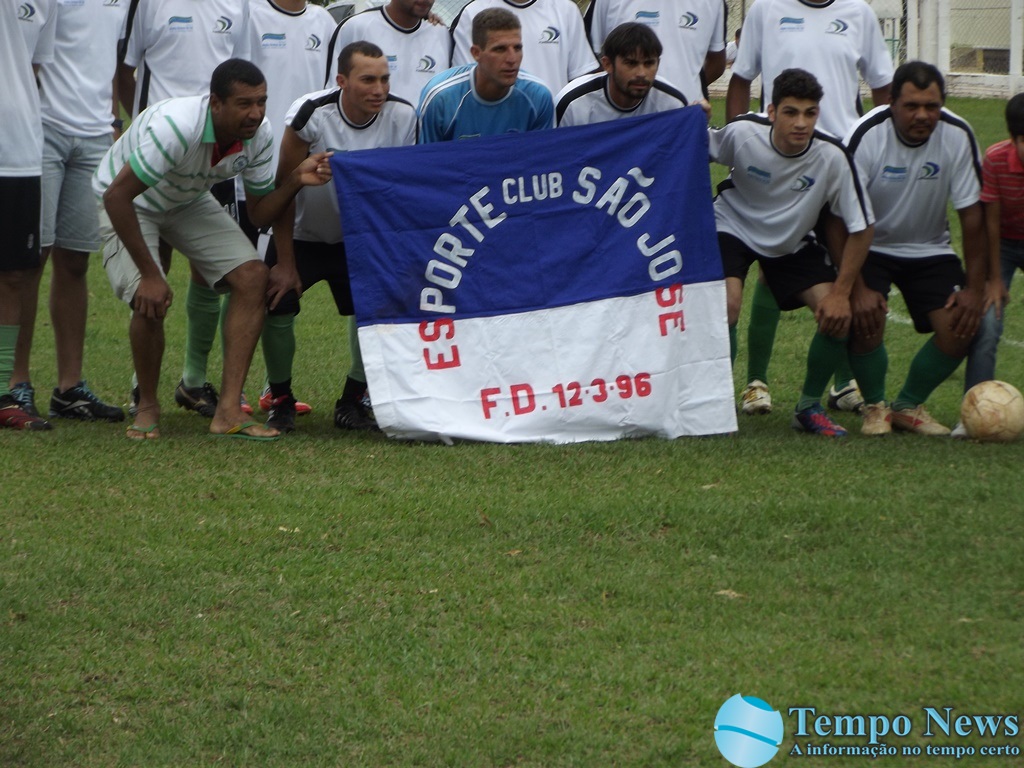This photo captures a team of the Esporte Club São Jose FD 12396, presumably a Brazilian soccer team, posing on a grassy field. The team members are arranged with the front row squatting and the back row standing, although the heads of the back row players are cropped out of the frame. The players are donned in white jerseys with a black stripe down the shoulder and sleeve, paired with black shorts and green socks. In the center stands a goalie distinguishable by his blue teal shirt. On the left side of the front row, there's an individual, possibly a coach, wearing khaki shorts, flip-flops, and a green-and-white striped polo. The front row players are holding a banner that is blue on the top and white on the bottom, emblazoned with the words “Esporte Club São Jose FD 12396” in red and white lettering. A soccer ball is placed on the ground near one of the team members. In the lower right corner of the photo, there is a watermark with the Tempo News logo along with the text “Tempo News e Informação Tempo Certo.” The blurred background hints at chairs or a gate. Some players are wearing cleats, while others sport sandals, emphasizing the casual nature of the photo shoot.